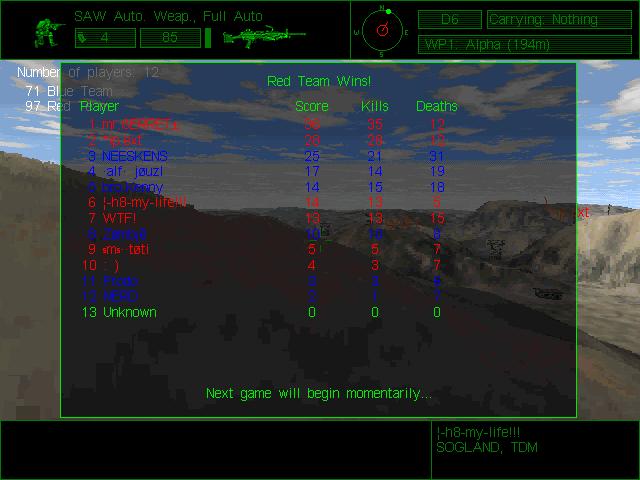The image depicts a video game screen with a detailed scoreboard overlay. At the top, there is a black strip with a small yellow soldier icon next to text that reads "SAW, Auto Weapon, Full Auto," accompanied by an illustration of a gun. The screen also shows directional indicators like "D6". The game background features a desert-like, mountainous terrain with visible sand and rocks, viewed through a transparent overlay net. In the upper left corner, it indicates the number of players, which is 12. The blue team has a score of 71, while the red team, which has won, has a score of 97, as noted in green text at the top center of the screen. The scoreboard details individual player statistics, including scores, kills, and deaths, displayed in red and blue text matching each team. At the bottom of the screen, a message in green text states, "The next game will begin momentarily."